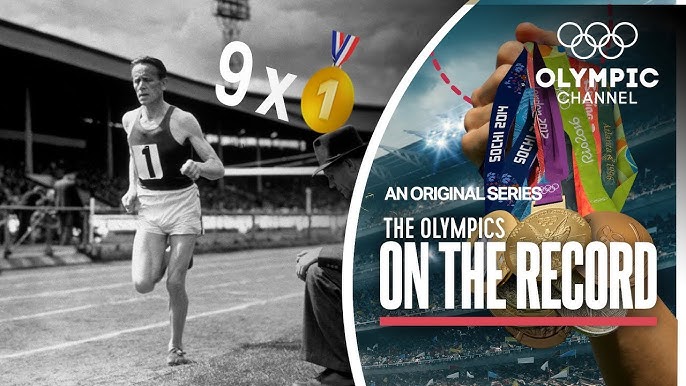The image is an Olympic advertisement poster divided into two contrasting halves by a white curved line. The left-hand side features a nostalgic black-and-white photograph from the 1940s or 1950s of a runner on a track. This athlete, wearing white shorts and a dark tank top with a paper bib number 1, appears to be a long-distance runner, given his muscular legs and composed form. The background reveals a railing next to the track and some makeshift shelters, possibly seating or other structures.

In contrast, the right-hand side bursts with vibrant colors and modern imagery. A hand clasps multiple colorful Olympic medals adorned with ribbons in hues of blue, purple, lime green, and orange, with 'Sochi 2014' inscribed on them. Above this, the iconic five interlocked Olympic rings and the words "Olympic Channel" are prominently displayed. Below, it advertises "An Original Series: The Olympics on the Record" in white text, emphasizing a historical narrative of Olympic achievements.